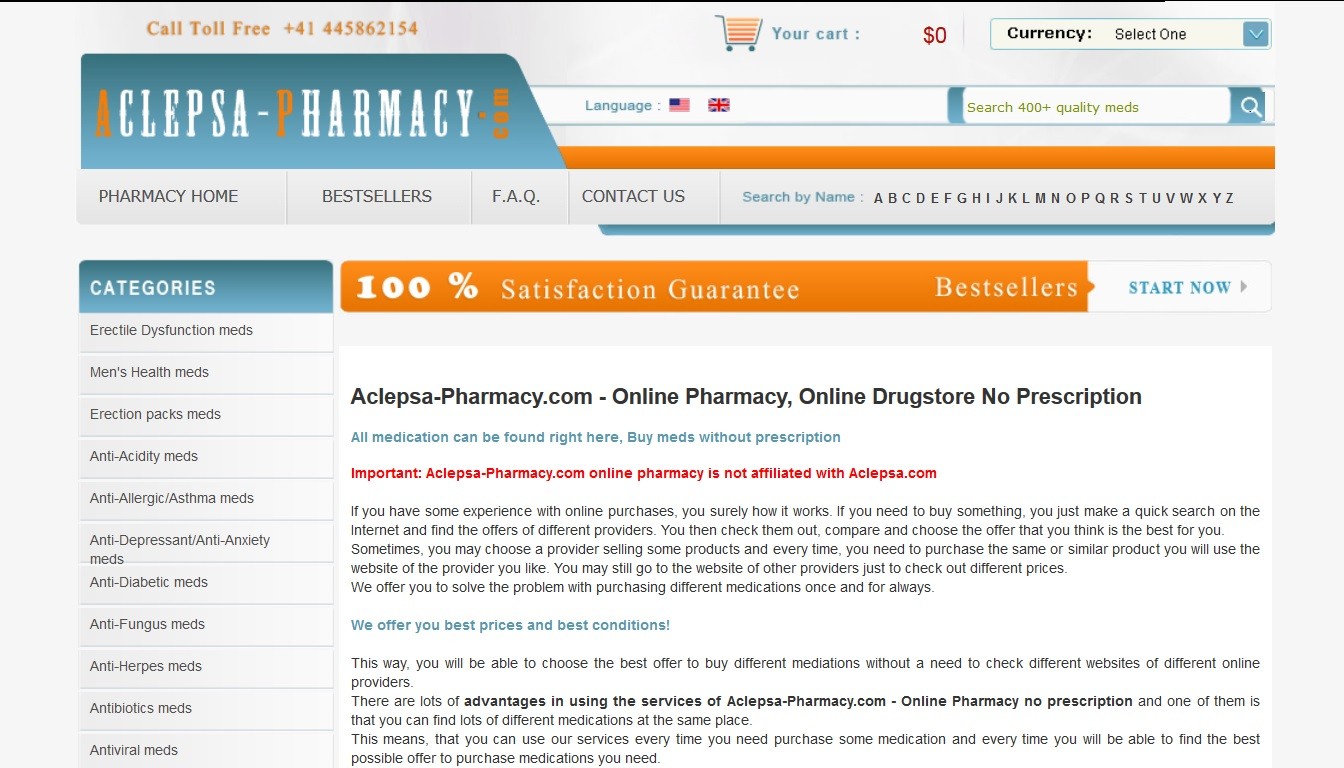**Image Caption:**

The image features a call to action for a pharmacy, highlighting various aspects and services. At the top, a toll-free number is prominently displayed as 411-445-8686, followed by an additional number, 214. Below this, there's a large blue tab with the text "Eclipsa-Pharmacy.com" where the letters 'a' in Eclipsa and 'P' in Pharmacy are in orange, while the rest of the text remains white. Interestingly, the "dot" in ".com" appears as a floating orange dot adjacent to the 'y' in Pharmacy, with a comma placed sideways to its right.

Above the main content area is a card section showing a zero-dollar balance with options to select different currencies. Users have the capability to conduct searches and change the language settings, with options currently available for the United States and the United Kingdom.

Just below the blue tab, and to the left, there are navigational links in capital letters: PHARMACY HOME, BESTSELLER, FAQ, CONTACT US, and SEARCH BY NAME A-Z. Adjacent to these links on the left are tabs for various categories such as ED Meds, Men's Health, Erectile Packs, Anti-Acidity, Anti-Allergic, Asthma Meds, Antidepressants, Diabetic, Fungus, Herpes, Antibiotics, and Antiviral medications.

To the right side of the image is a bold statement indicating that this is an online, no-prescription-needed drugstore. It emphasizes that all medications can be purchased without a prescription and highlights that this site is not affiliated with Eclipsa.com. 

Additionally, there is important information in red, detailing that you can expect the best prices and conditions, and the convenience of not needing a prescription, which enhances its appeal. Despite not being affiliated with the original Eclipsa site, it markets itself as a reliable and affordable alternative for medication.